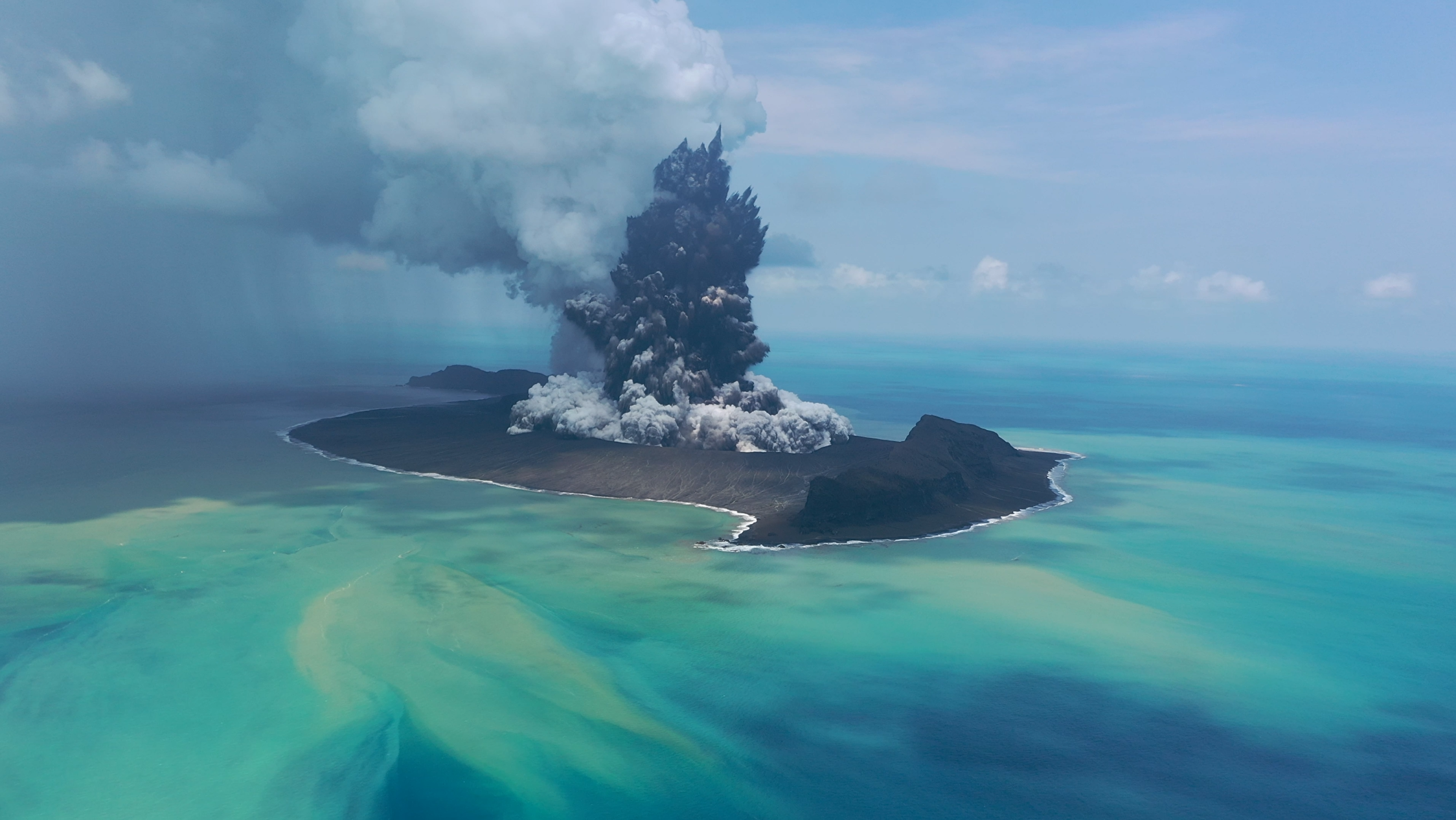The image showcases a small island in the middle of a calm ocean, with water exhibiting shades of bluish-green and deep blue. The island, shaped somewhat like a badge, features a dark brown structure that emits a white cloud of smoke, suggesting a volcanic eruption. The sky overhead is a soft light blue, dotted with numerous clouds, blending with the smoke from the eruption. The scene appears tranquil and surreal, with very still and smooth waters surrounding the island, adding an otherworldly or even science fiction-like quality to the landscape.